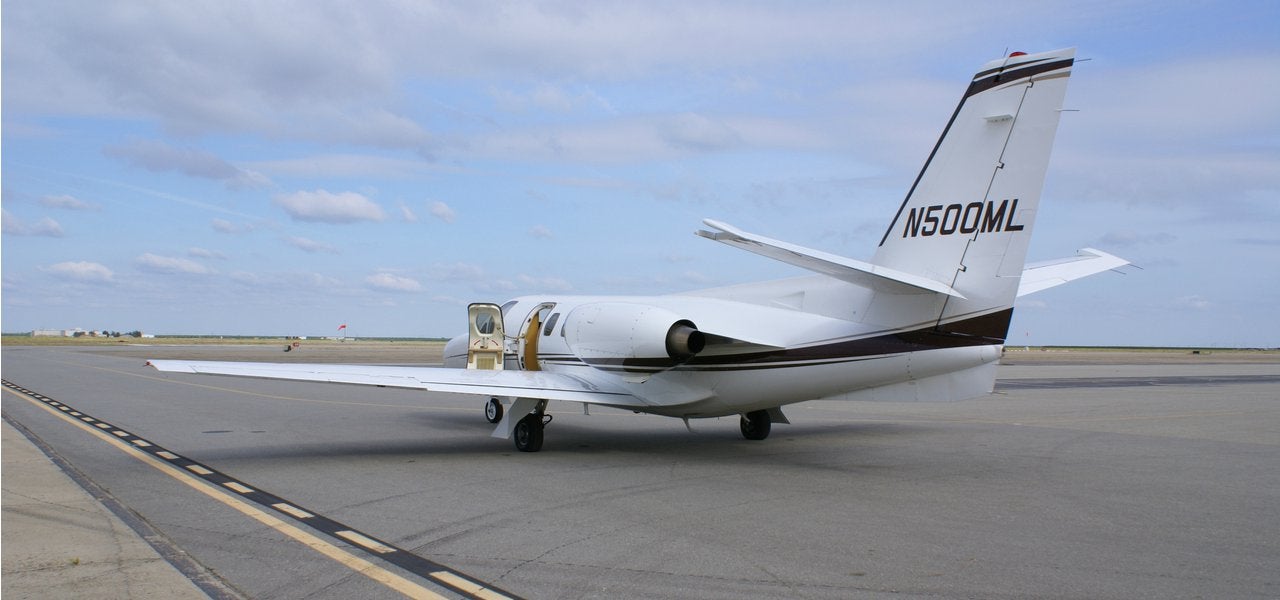The image captures a private jet positioned on a runway. The jet, sleek and white, features distinct navy and black pinstriping down its side and along the top of its tail, marked with the code N500ML. The plane’s open cockpit door reveals a cream-colored interior. A single large jet engine is visible on the left side of the aircraft. The runway itself stretches from the lower right to the upper left of the image, adorned with black and yellow stripes and tire marks, signaling frequent use. The horizon line bisects the picture, showcasing a pale blue, overcast sky filled with fluffy white clouds. In the distance, a small red flag can be seen against the wide-open backdrop, reinforcing the sense of space and openness. The lack of direct sunlight further accentuates the overall overcast ambiance.